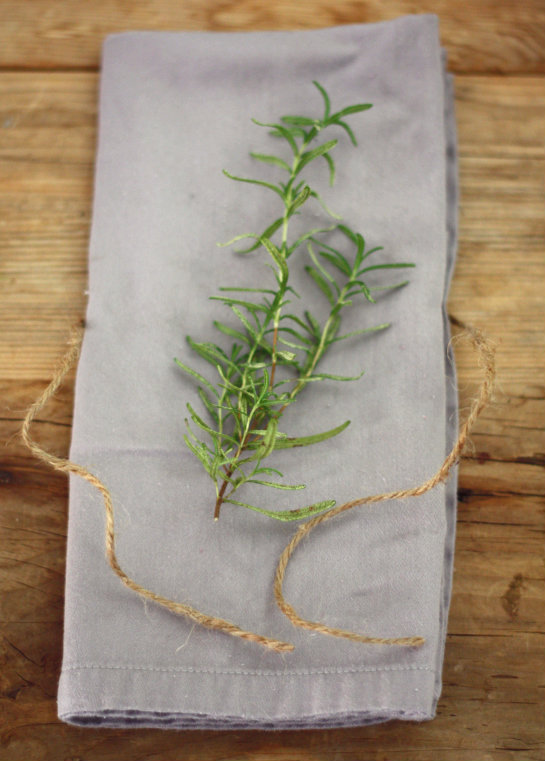This up-close photograph captures several stems of green rosemary arranged on a folded napkin laid on a light wooden table, which appears to be made from assembled wooden planks. The rosemary, identifiable by its long, narrow, and pointy leaves, is splayed out atop the napkin, which is either a shade of lavender or light blue. The napkin seems to have been initially tied with twine, which is now untied and visible on either side, suggesting it might have served as a pouch for the herbs. The composition provides an intimate view of the fresh, fragrant foliage against the rustic backdrop of the wooden surface.